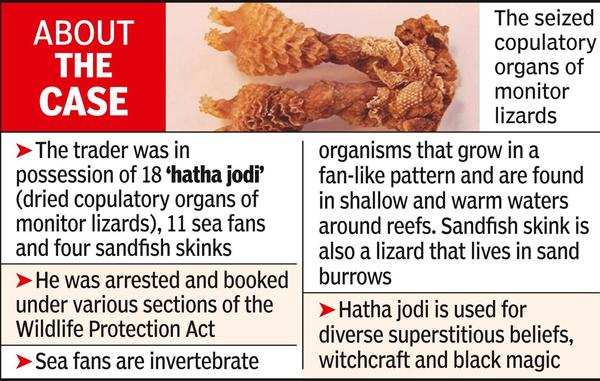This image depicts a summary of a wildlife trafficking case, featuring a mix of text and a photograph on a red background. The upper left corner states "About the Case," highlighting that an individual was arrested for illegal possession of wildlife items. Specifically, the person was found with 18 Hatha Jodi, dried copulatory organs of monitor lizards, 11 sea fans, and four sandfish skinks. These items were seized and the individual was booked under various sections of the Wildlife Protection Act. The image provides additional details, explaining that sea fans are invertebrate organisms that grow in fan-like patterns in shallow, warm waters near reefs, while sandfish skinks are lizards that inhabit sand burrows. Furthermore, Hatha Jodi is noted for its use in superstitious practices, witchcraft, and black magic.